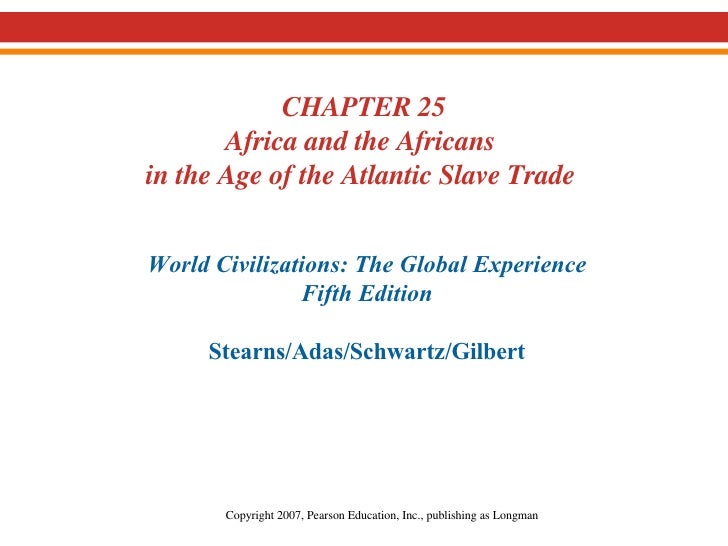The image is a square representation of the beginning of Chapter 25 from an educational website. It features plain text over a white background and appears to be part of a slide or digital presentation. At the top, there is a burgundy line stretching horizontally across the page, followed by a thinner orange line directly beneath it. Centered below these lines, in larger burgundy text, is the chapter title: "Chapter 25, Africa and the Africans in the Age of the Atlantic Slave Trade." Below the title, in blue text, are the details of the book: "World Civilizations: The Global Experience, 5th edition," along with the authors' names: Stearns, Adas, Schwartz, and Gilbert. At the bottom, in small black text, is the copyright information: "Copyright 2007, Pearson Education, Inc. Publishing as Longman." The entire layout is upright with all text horizontally aligned in a straightforward, academic style.